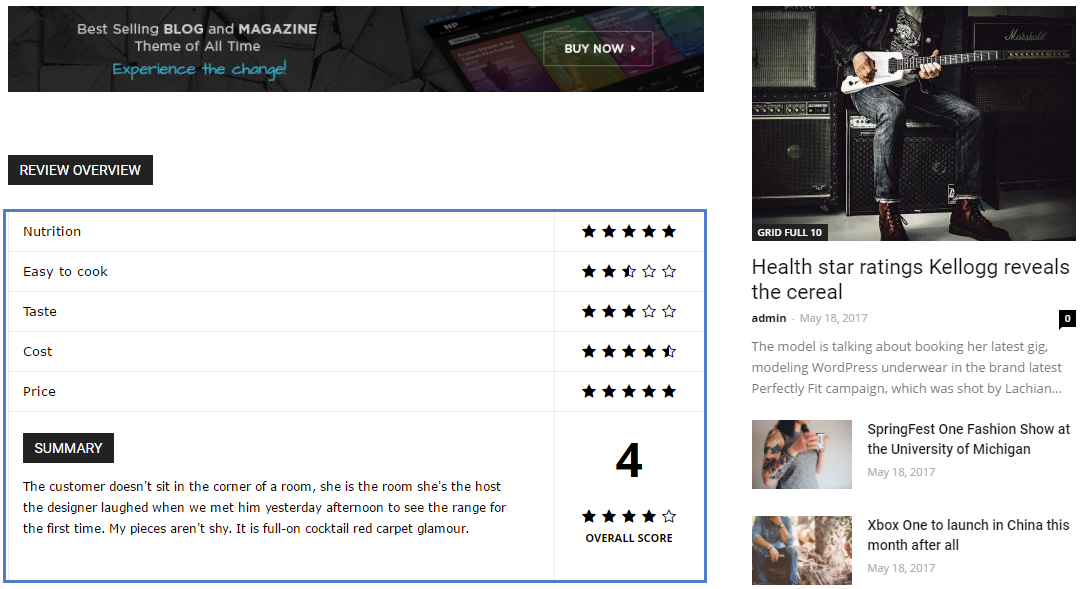This image is a detailed screenshot from a website, which appears to be a sales page for a WordPress theme, focusing on a blog and magazine template. The left side features a grayed-out photo, which serves as a dark gray rectangular header. Next to this, on the right side of the small rectangle, there is what looks like a screenshot displaying a list of potential magazine titles.

Prominently, on the left side of the screenshot, there is a headline that reads, "Best-selling Blog and Magazine Theme of All Time - Experience the Change." This strongly suggests that the page is advertising a particular WordPress theme.

Taking up about half the page and situated halfway down, there is a white rectangle bordered by a medium blue line. Inside this rectangle is a table resembling something typically seen on a blog, containing a list of items: Nutrition, Ease of Cook, Taste, Cost, and Price. To the right of each item, there are star ratings provided, giving a sense of evaluation or review.

Below this table, there is a summary section filled with placeholder, nonsensical text often used in web templates to indicate where content will be placed. The ratings within the table do not necessarily hold any actual significance and are likely part of the template's demo content.

On the right-hand side of the image, there is a stock photograph of a person playing a bass guitar, shown from below the shoulders down to the legs. The individual appears to be a man dressed in dark blue jeans and brown work boots. Below this photograph, there are some smaller headlines and snippets of text, along with a couple of small images and accompanying headlines, adding further content layout examples.

Overall, this image presents a polished example of a web template designed for a magazine and blog theme, showcasing various possible elements such as headers, star-rated tables, stock images, and formatted text to give potential buyers a clear idea of the theme's capabilities.